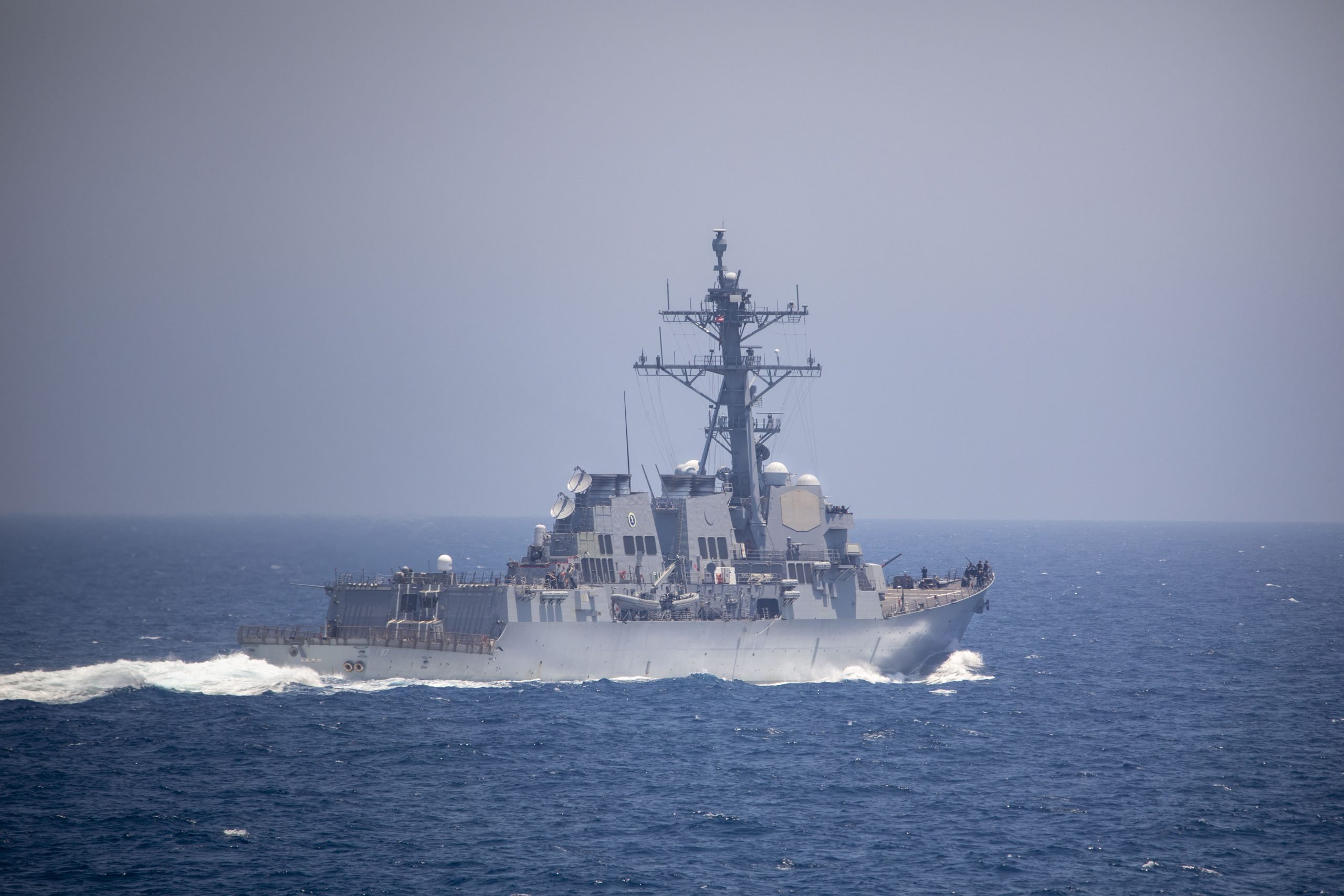This color photograph, taken in landscape orientation, captures a steely gray military naval warship as it sails through the calm, deep blue waters of the open ocean, with no land in sight. The vessel, prominently positioned in the center of the frame, has its bow pointed to the right and stern to the left, cutting through the water and creating a wake of white foam behind it. A large mast towers over the deck, adorned with an array of electronic gear, antennas, satellite dishes, and radar domes aimed in various directions. Toward the front of the ship, a gun turret is prominently visible. Additional equipment lines the deck's border, hinting at the ship's complex functionality. Despite the sun's presence, the sky is a dull, misty gray, casting a somber, monochromatic palette over the scene, which captures a realistic and detailed representation of naval maritime power.